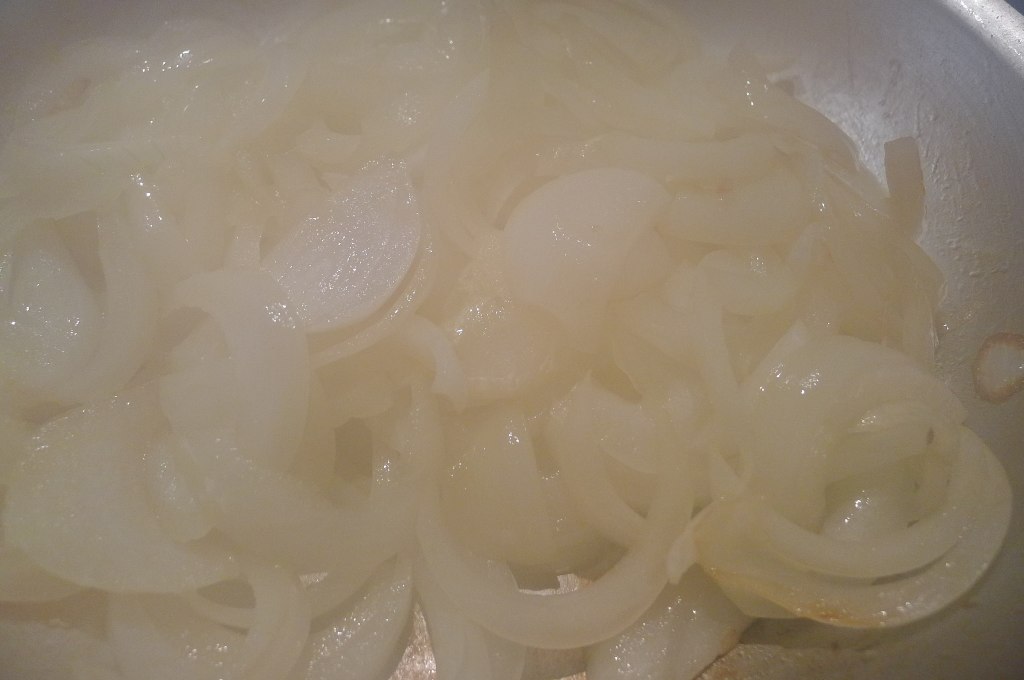This image features a shallow, silver pan, possibly a skillet, containing slices of onions that appear to have been cooked. The pan is identifiable by a small round rivet where a handle would typically be attached. Inside the pan, the onions are sliced into medium thickness, with some pieces being wedge-shaped from the center section of the onion. The onions exhibit a slightly yellowish hue with a shiny, dewy appearance, suggesting they have been either sautéed or are in the process of cooking. A few pieces show browning at the edges, indicating they are beginning to caramelize. One can observe some steam rising from the upper left corner of the image and reflections of light glistening off the onion slices. The background features a small black surface, providing contrast to the glossy, off-white onions and the metallic sheen of the pan.